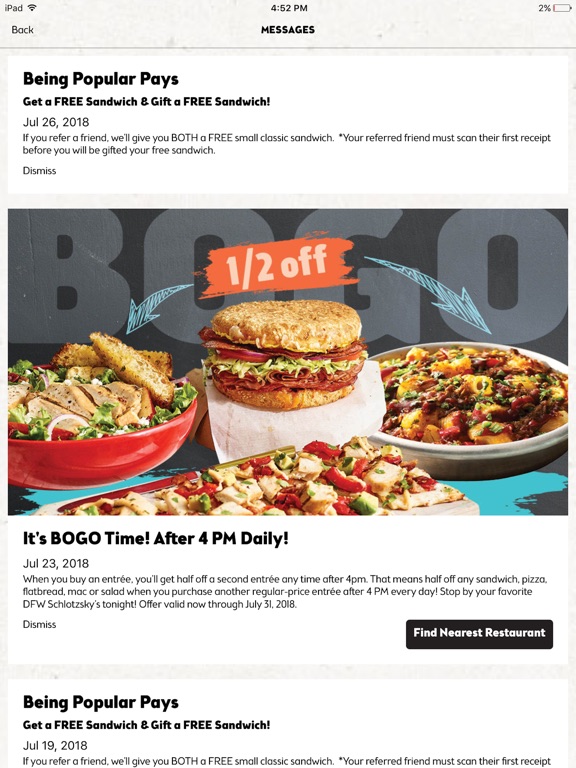The iPad screenshot captures a page from a restaurant's application, specifically the messages section. In the upper-left corner, "iPad" is visible, indicating the device in use. The screen title "Messages" is prominently displayed at the top, with a back button located to the left. Several promotional messages are listed:

1. The first message reads "Being popular pays: Get a free sandwich and gift a free sandwich," dated July 26, 2018. It offers more information on this deal, aiming to reward customers for their referrals.

2. A large banner image follows, showcasing four different meal options over a background that spells "BOGO" in large letters. Blue, hand-drawn arrows point to two of the meals, with a "one-half off" label between them. The message title announces, "Buy One Get One Off BOGO Time," available after 4 PM daily from July 23, 2018. A button on the right-hand side allows users to find the nearest restaurant. Below this information, there is an option to dismiss the message.

3. The final visible message repeats the promotion "Being popular pays: Get a free sandwich and gift a free sandwich," but is dated July 19, 2018. It explains a referral program where referring a friend grants both the referrer and the referee a free small classic sandwich.

Each promotional message has an option to be dismissed by the user.